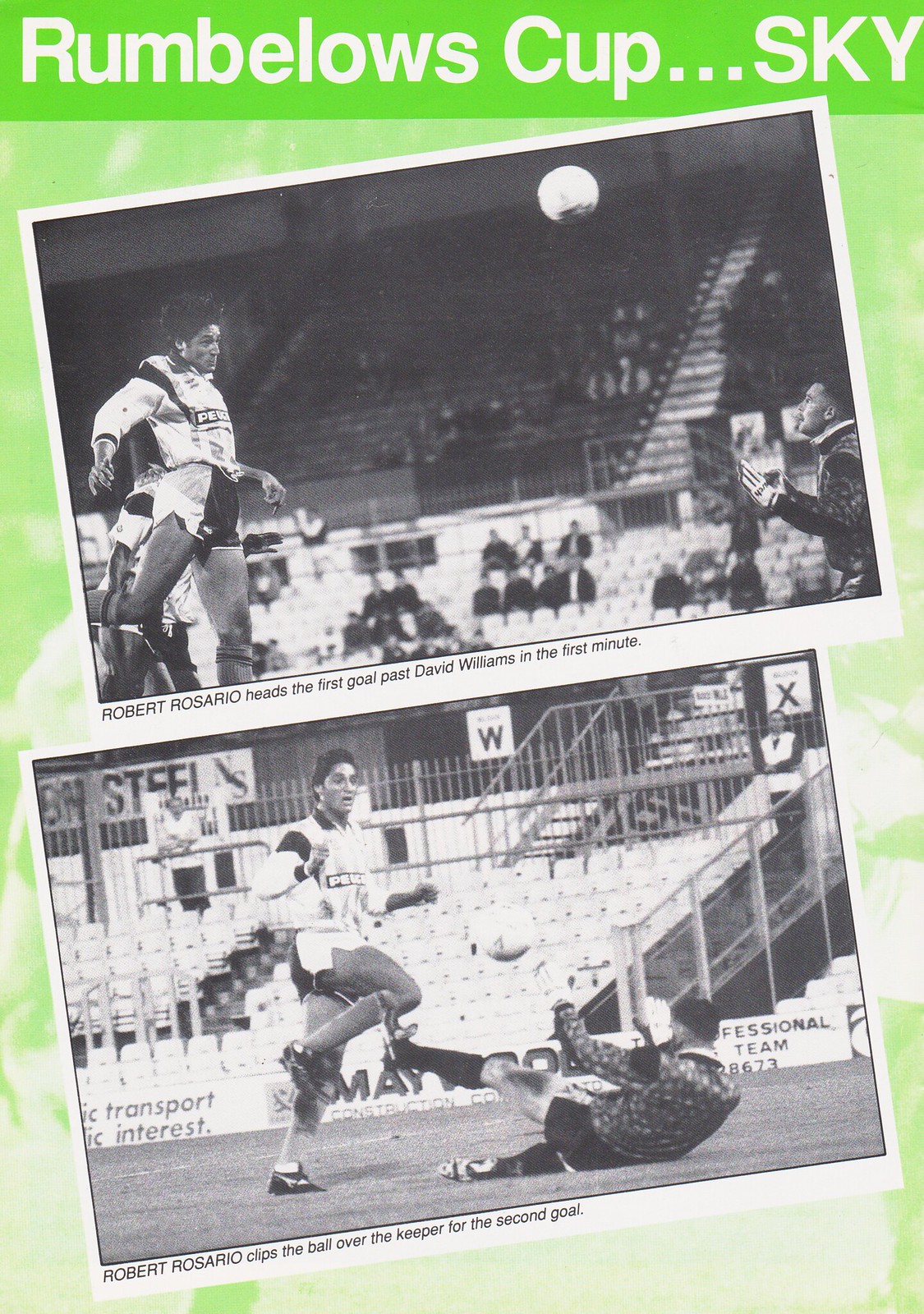The image is a vintage soccer program poster with a dark green background at the top. Prominently, it features the text "RUMBLOWS CUP... SKY" in large, white, uppercase letters. Below this heading, there are two angled black-and-white photographs depicting crucial moments from a soccer match.

In the first photograph, Robert Rosario is seen leaping into the air, his face scrunched with concentration as he heads a soccer ball past the goalkeeper, David Williams, during the first minute of the game. The goalie is in the right corner, his hands outstretched toward the ball. This image is captioned, "Robert Rosario heads the first goal past David Williams in the first minute."

The second photograph captures another action moment: Robert Rosario is running to the left, with his right leg bent and his arms straight beside him. In the background, white-colored bleachers are visible. On the ground, a player—presumably the goalie—has his right leg in the air and arms stretched upwards, his body partially lifted off the ground. The caption reads, "Robert Rosario clips the ball over the keeper for the second goal."

Together, these elements create a detailed narrative of Rosario's significant contributions to the match, vividly illustrated and captioned on this nostalgic poster.